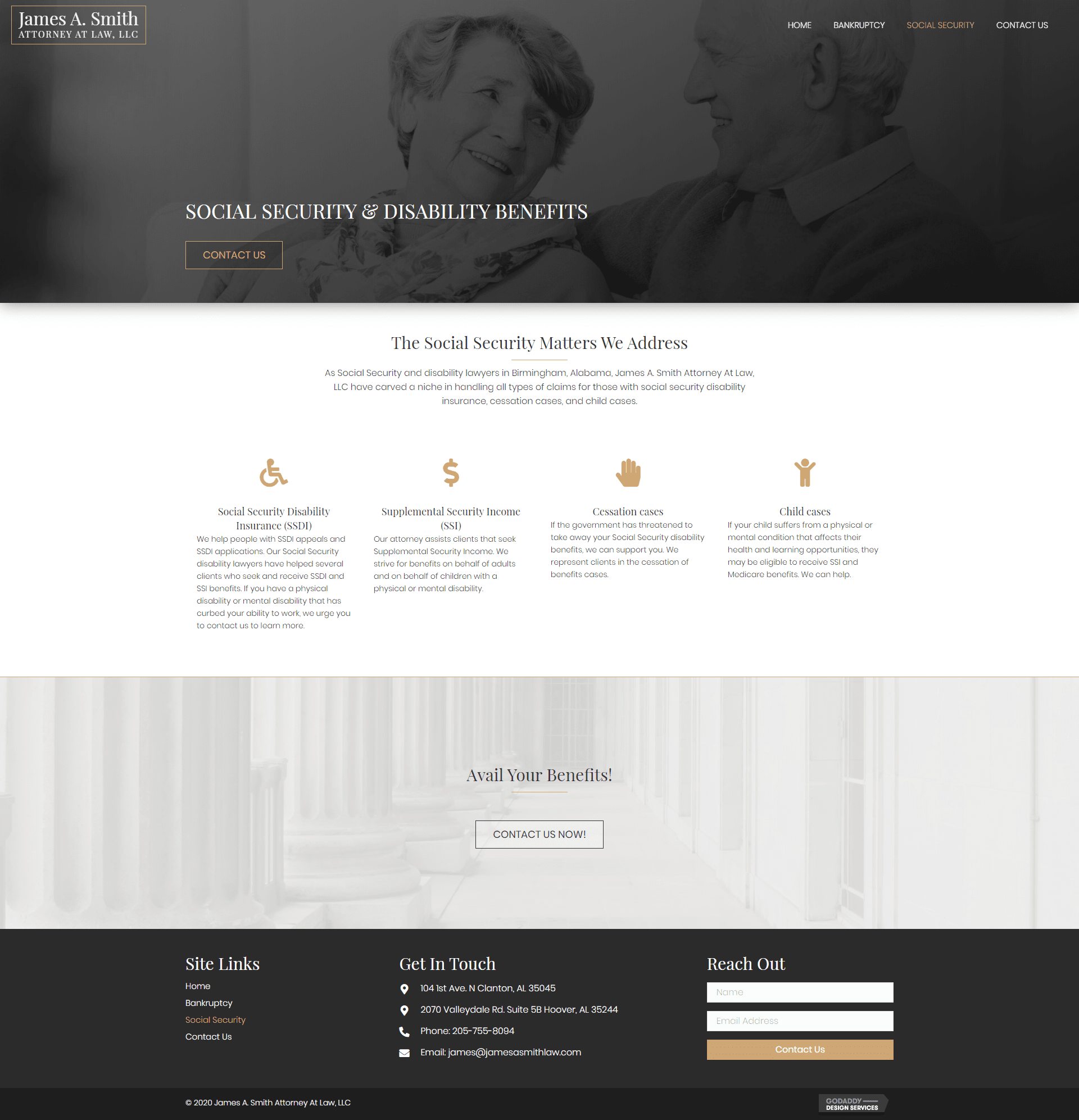**Screenshot of a Legal Services Website**

The screenshot showcases a website for James A. Smith, Attorney-at-Law, LLC. The top left corner features the name "James A. Smith, Attorney-at-Law, LLC" in white text. The background consists of a darkened banner image of an elderly couple, with the woman having short hair looking lovingly at the man, who is reciprocating with a tender gaze. This image captures them from the chest up.

Towards the upper right-hand corner, there is a navigation menu with options labeled "Home," "Bankruptcy," "Social Security," and "Contact Us." The "Social Security" option stands out in yellow, while the others are in white.

Beneath the woman's chin in the picture, a bold headline in all caps reads, "SOCIAL SECURITY AND DISABILITY BENEFITS," followed by an orange "Contact Us" button. Below this section is the text "The Social Security matters we address" centered in the middle, along with three lines of smaller text that are too blurred to read.

Four gold-colored icons representing different aspects of social security benefits are displayed horizontally. These icons include a wheelchair, a dollar sign, a hand, and a person's body. Beneath these icons, the text "Avail Your Benefits" appears on a white background that is slightly faded, suggesting an interior setting with curtains and windows in the backdrop.

Another "Contact Us Now" button, outlined in black, is located below this section. The lower portion of the webpage includes a black section labeled "Site Links" with four listed items and a "Get in Touch" section with four corresponding icons, though the text is too small to read.

On the right side of this part, there is a "Reach Out" section in white text, accompanied by two input boxes for user information, followed by a yellow "Contact Us" button beneath it. Additional text and labels are present at the bottom left and right sides, but the details are not legible in the screenshot.